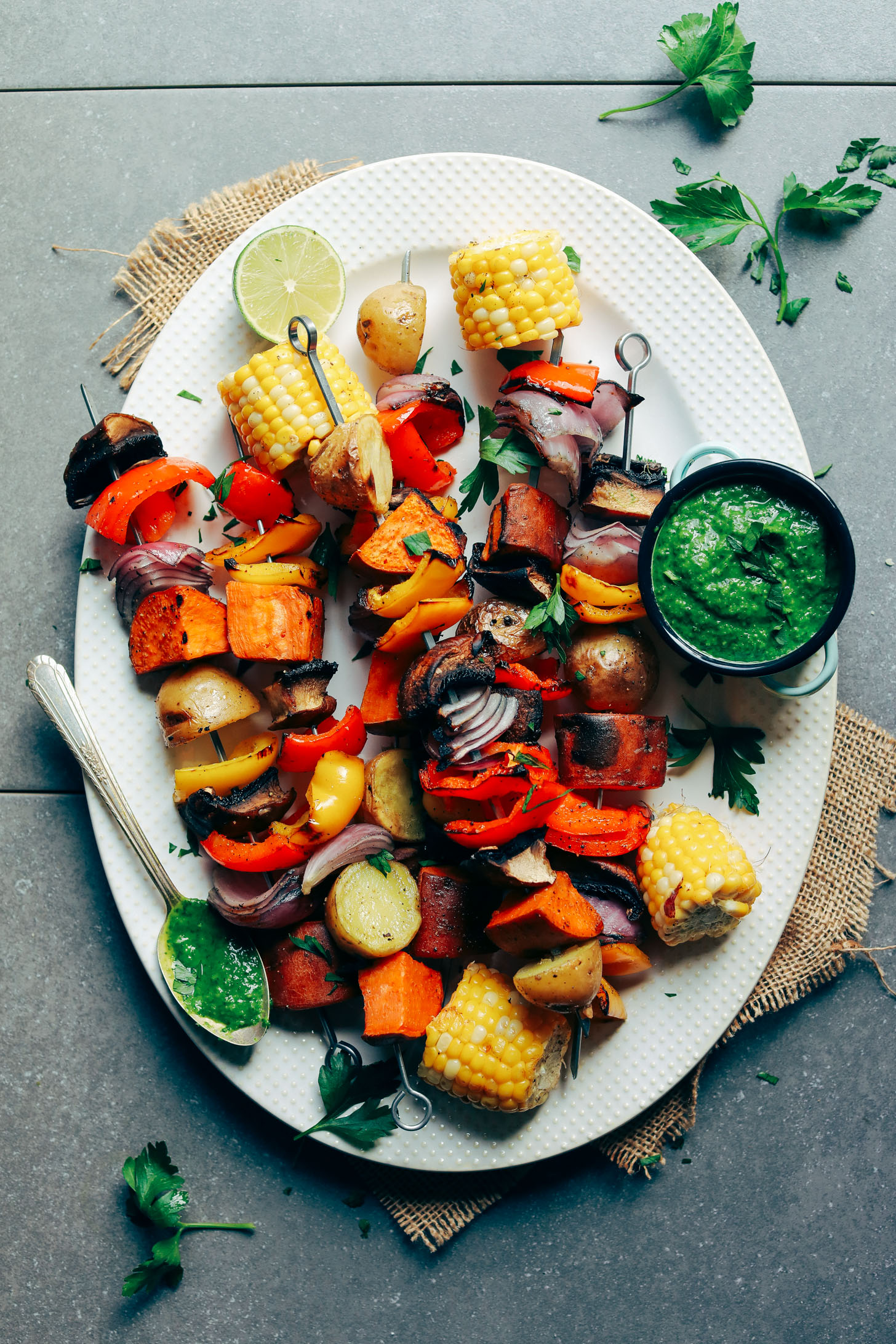This is an indoor, close-up photograph of an artistic and vibrant plate of skewered kebabs brimming with a medley of vegetables and meat. The large, oval white serving plate prominently displays six metal skewers laden with chunks of colorful bell peppers, onions, carrots, corn on the cob, potatoes, and meat. To the right of the plate sits a small metal pot filled with a green sauce, possibly chimichurri, with a silver spoon dipped in the sauce resting nearby, indicating it has been recently used. The plate rests on a burlap cloth, adding a rustic touch to the composition. Strewn around the plate are loose vegetables and sprigs of cilantro, enhancing the artistic presentation. The setting appears to be on a slate or cement-like table, contributing to the photograph's stylish and inviting appeal, aimed at enticing one to enjoy the flavorful feast.